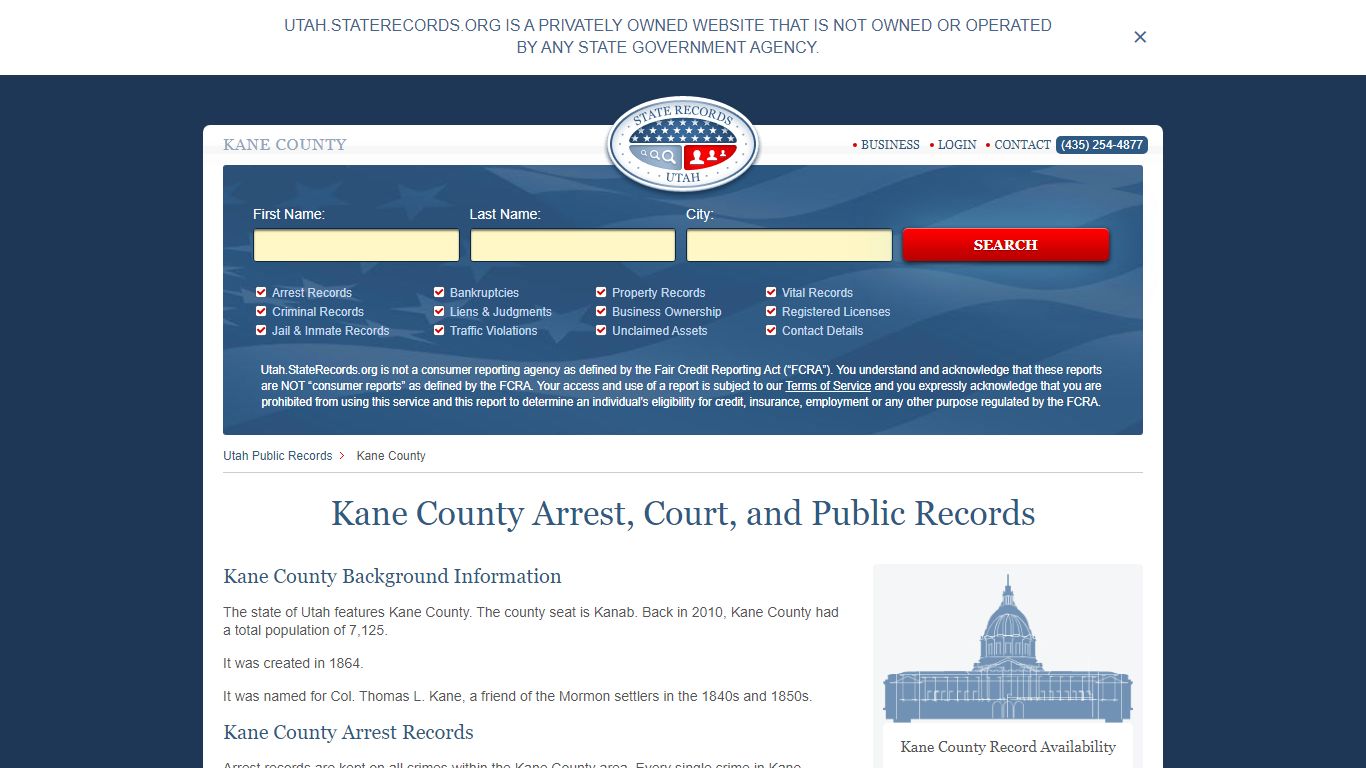The webpage for UtahStateRecords.org, a privately owned website unaffiliated with any state government agency, features a prominent header with this disclaimer. Below the header, the page has a navy blue background with an image that is slightly obscured. At the top of the page, "Kane County" is prominently displayed, followed by the phrase "State Records of Utah" with a small symbol in between. The navigation options include links for business logins, contact information, and an additional blue-tabbed link that is indistinguishable.

The website offers a search function where users can input a first name, last name, and city to look up specific records. Various checkboxes below the search fields delineate the kinds of records that can be searched. Immediately beneath this search section, the page displays information specific to Kane County, emphasizing "Utah Public Records / Kane County" and "Kane County Arrest, Court, and Public Records."

Further down, there is a detailed section on Kane County, including background information such as the location of the county seat in Kanab and historical details about its establishment. The page concludes with a section titled "Kane County Records," although the specifics of the records in this section are not visible from the provided description.